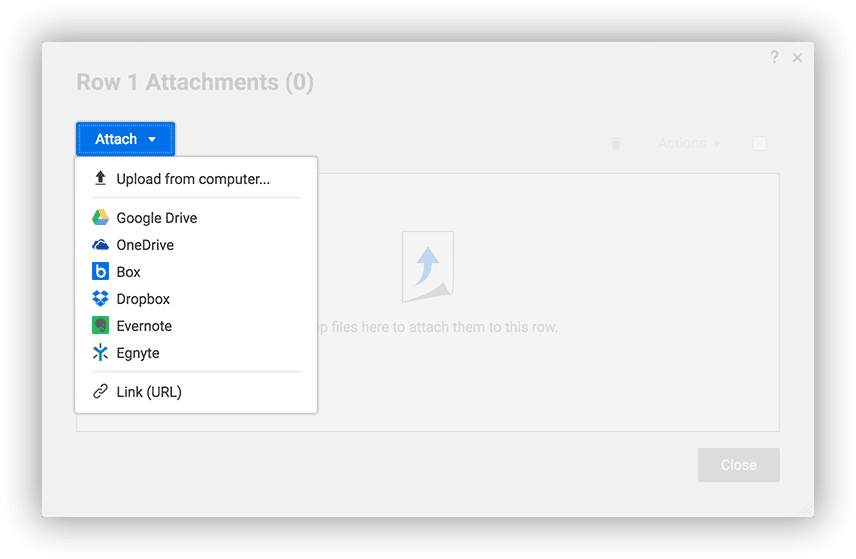This detailed caption describes a screen capture of a file attachment interface on a computer:

The image is a horizontal screenshot, seemingly taken from a desktop or laptop computer, bordered by a shadowy, medium-gray box that casts a faint shadow around it. In the top-left corner of the interface, a label reads "Row 1, attachments (0)" in a different shade of gray. On the top-right corner, there are two icons: a question mark and an "X".

To the left, below the label, there is a blue rectangular button with white "Attach" text and a downward-pointing white arrow. Upon clicking this button, a dropdown menu appears. This menu includes options for file attachment, each with a colorful icon and black text: "Upload from computer," "Google Drive," "OneDrive," "Box," "Dropbox," "Evernote," "Genite," and "Link URL."

In the center of the screenshot, there is a rectangular area with a large blue upward-pointing arrow, suggesting where files should be dragged to attach them. However, the view is partially obscured by overlapping interface elements, leaving only partially visible instructions: "drag files here to attach them."

Lastly, at the bottom-right of this rectangular area, there is a dark gray "Close" button, which appears to be inactive or unclickable at the moment of capture.